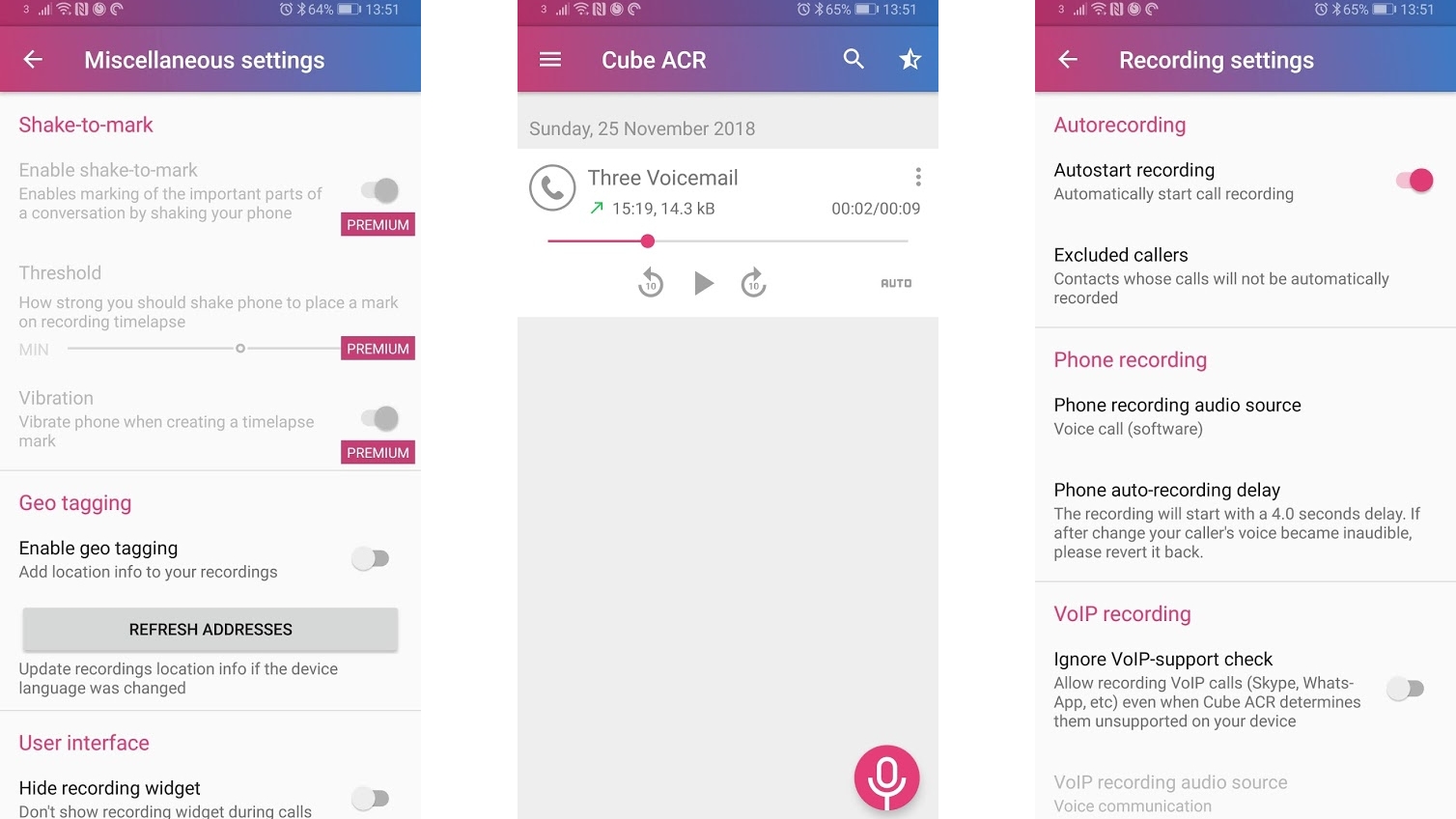This series of three screenshots features distinct, informative interfaces centered around a common theme, adorned with a visually striking pink-to-bluish purple ombre bar at the top. Each screenshot is hosted in this gradient header which varies seamlessly across the set.

The first screenshot is titled "Miscellaneous Settings" within this vibrant bar. Prominently displayed in pink font is the feature "Shake to Mark." This setting is accompanied by a toggle switch, currently activated, allowing users to mark significant parts of conversations by shaking their phone. Below this is the "Premium" section, which includes multiple advanced settings:
- **Threshold**: This section specifies the intensity of the shake needed to mark recordings. It features a draggable adjustment bar. The "Premium" label in a pink box indicates that this functionality requires a premium subscription.
- **Vibration**: When enabled (as it is in this screenshot), the phone vibrates upon marking a segment of the recording. This setting is also marked as a premium feature.
- **Geotagging**: This option, which toggles the addition of location data to recordings, includes additional buttons for refreshing the address and controlling related settings. 

Other items include "User Interface" options, which incorporate features like hiding the recording widget.

The second screenshot features the heading "Cube ACR" in the same colorful bar, highlighting a section dedicated to managing "Voicemail." This likely includes options to listen, save, or delete voicemails directly from the interface.

In the third and final screenshot, the title in the color bar changes to "Recording Settings." Key settings shown here include:
- **Auto Recording**: This possibly refers to automatically recording selected conversations.
- **VOIP Recording**: This suggests options for recording VOIP (Voice Over Internet Protocol) calls.

These detailed screenshots collectively emphasize the user's control over various advanced settings, ensuring a customized recording and marking experience.